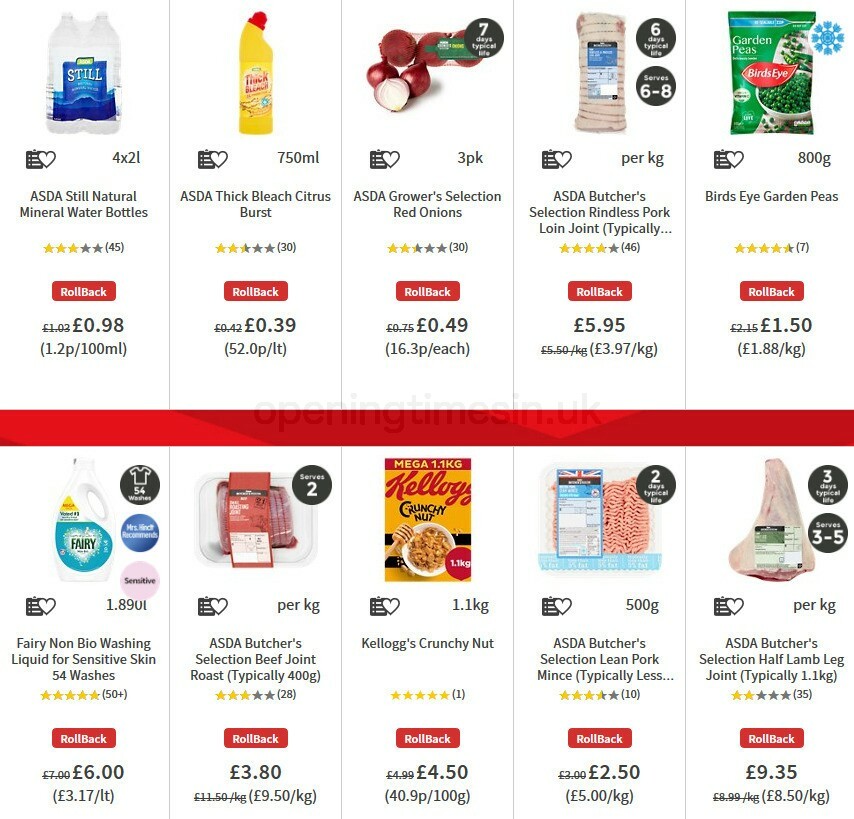This screenshot is from a shopping listing on what appears to be a Walmart-like retail website, potentially ASDA. The page is organized into two rows, each showcasing five distinct items with accompanying photographs. The layout is separated by a prominent red bar running across the center of the page.

**Top Row:**
1. ASDA Still Natural Mineral Water Bottles - £0.98
2. ASDA Thick Bleach Citrus Burst - £0.39
3. ASDA Growers Selection Red Onions - £0.49
4. ASDA Butchers Selection Wranglers Pork Loin Joint - £5.95
5. Bird's Eye Garden Peas - £1.50

**Bottom Row:**
1. Fairy Non-Bio Washing Liquid for Sensitive Skin - £6.00
2. ASDA Butcher Selection Beef Joint Roast - £3.80
3. Kellogg's Crunchy Nut - £4.50
4. ASDA Butcher Selection Lean Pork Mince - £2.50
5. ASDA Butcher Selection Half Lamb Leg Joint - £9.35

This detailed and neatly-arranged shopping listing displays a variety of products ranging from groceries to household items, providing a comprehensive view for the shopper.